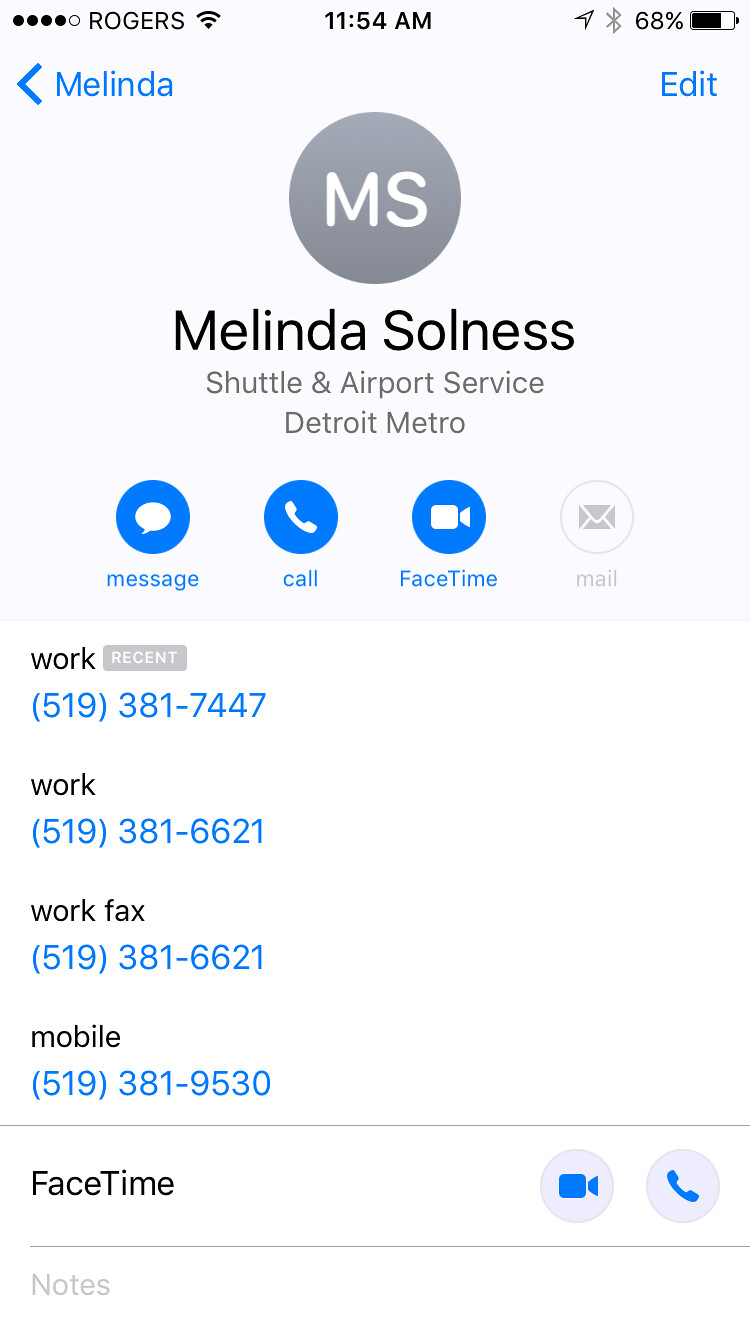The phone screen displayed detailed contact information for Melinda Solnys Shuttle and Airport Service, Detroit Metro. The screen showed multiple contact numbers including a primary work number, a secondary work number, a fax machine number, and a mobile number, all beginning with the area code 519 and prefix 381. Additionally, there was an option to initiate a FaceTime call. The contact information was accentuated in blue text set against a light blue and white background. The screen also provided real-time details such as the current time and the phone's battery percentage.